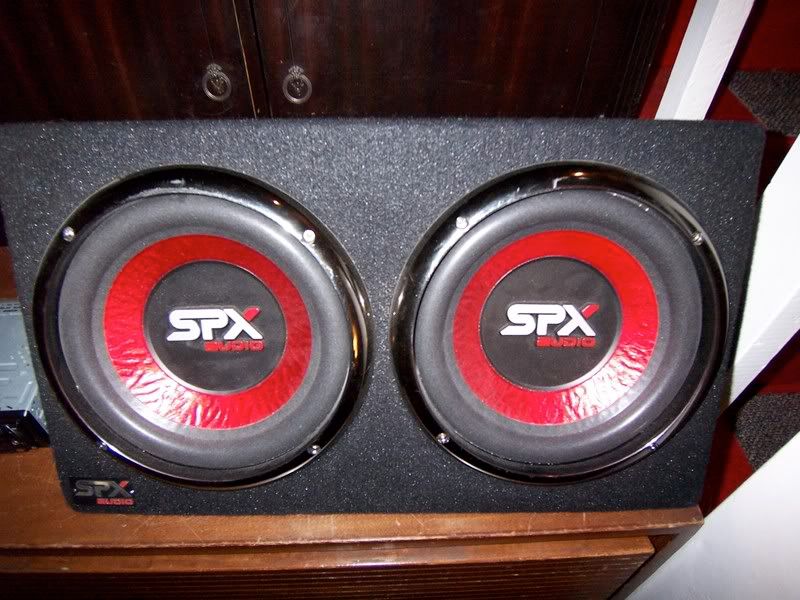The image prominently features a large, dark gray speaker box with a rough texture, centrally placed on a worn brown wooden table. The speaker system, branded as SPX Audio, consists of two speakers each distinguished by a shiny black trim, lighter matte black rims, and red circular accents. The letters SPX are boldly printed in white, with the top right tip of the X in red, and the text "audio" faintly visible below. Behind the table stands a darker wooden cabinet with circular metal knobs. Superimposed on the image is a semi-transparent circular watermark with the text "photobucket" in gray lowercase letters, followed by a gray strip with black lettering that reads "protect more of your memories for less," revealing it was uploaded via Photobucket. The setting suggests it might be in a privately owned space, potentially a bedroom.